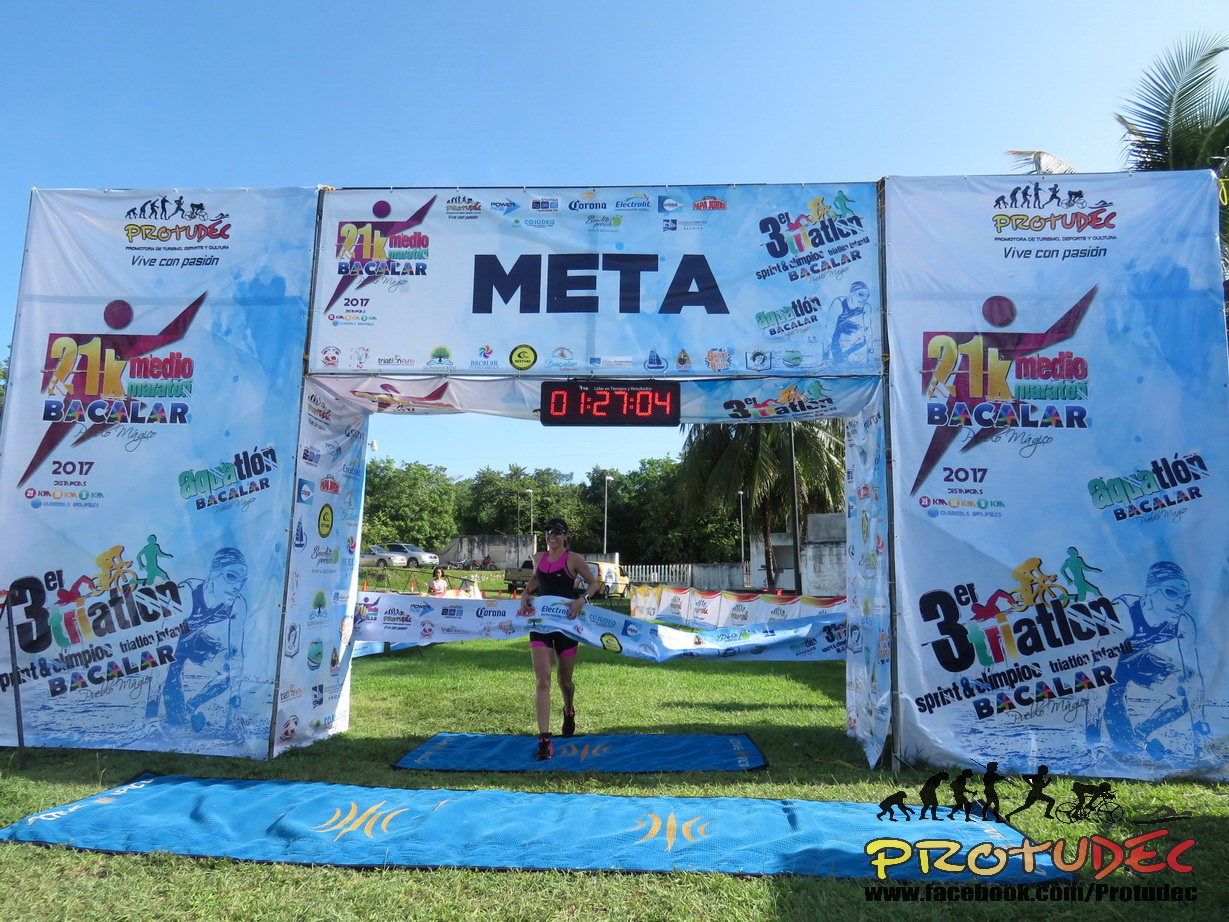The photograph captures the triumphant moment of a woman crossing the finish line of a triathlon race held in a park. The event appears to take place under a clear blue sky, with trees visible in the background. Central to the composition is an arch structure made from tent-like material, adorned with multiple illustrations and logos, including advertisements for Corona, Meta, and "21K." The arch is marked with the year 2017 and features vibrant designs, including illustrations of swimmers, suggesting the event's multifaceted nature involving swimming, cycling, and running.

The athlete, dressed in a black and purple spandex suit with pink accents, sunglasses, and a hat, is captured mid-stride as she breaks through the white banner at the finish line. Her hair is pulled back, and she has a joyful expression, indicating her victory. Below her feet lies a blue mat laid over green grass, solidifying the outdoor setting. Above her, a digital LED clock displays the race time: 1 hour, 27 minutes, and 4 seconds in red digits.

In the bottom right of the arch, a logo depicting the evolution of people with the text "Paitzo Tudak" is visible. The scene is lively with a few spectators in the background, adding to the celebratory atmosphere of this athletic accomplishment.